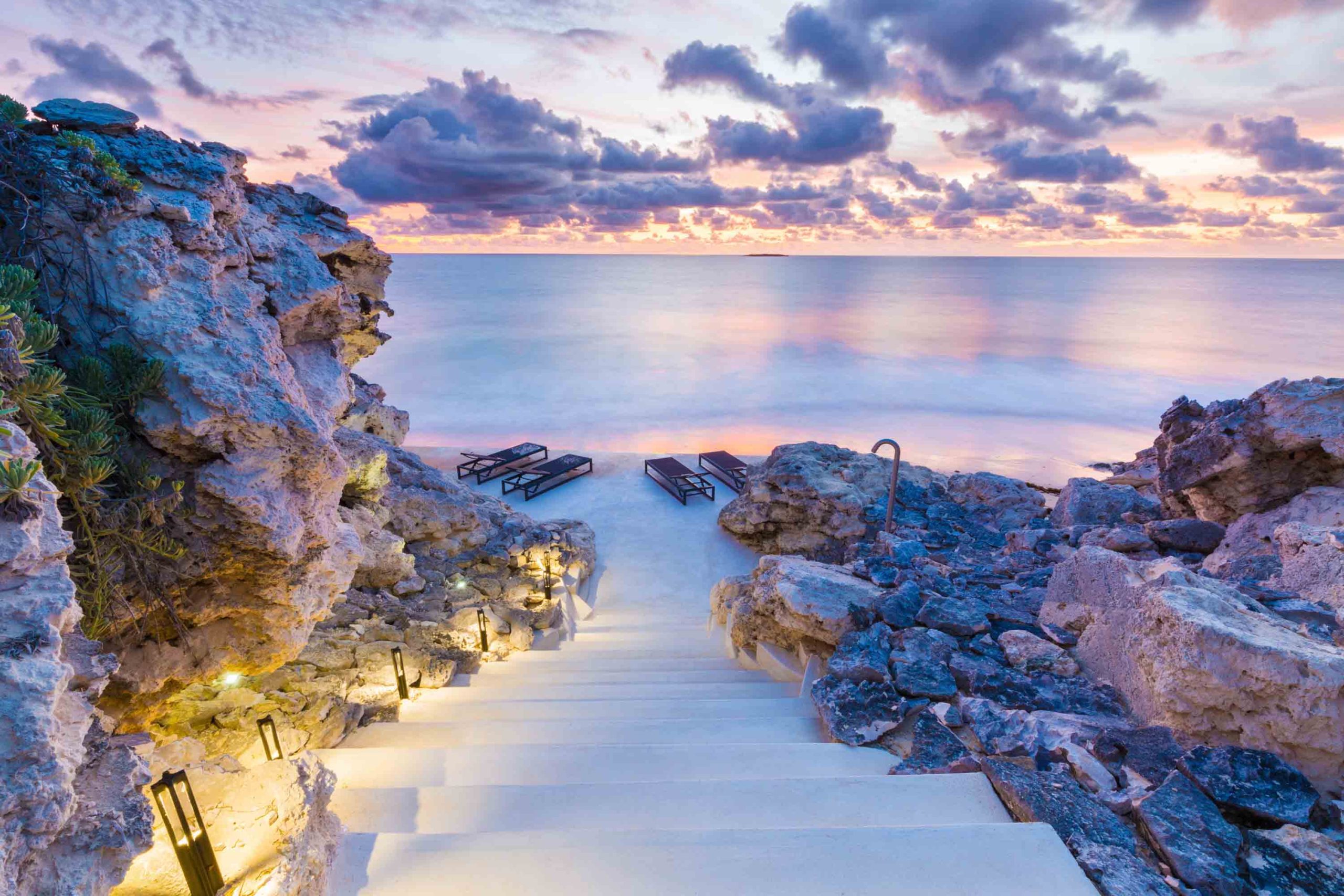The image captures a captivating seaside scene where a concrete stairway, illuminated by small lamps on either side, descends to a small beach area. The sky above is a blend of ominous dark gray clouds and softer, pink hues, giving the scene a surreal twilight quality. The ocean, reflecting the pink and white tones of the sky, features gentle waves crashing onto a sandy shore. On the left side of the stairs, a towering, rocky cliff dominates the view, whereas the right side showcases large rocks that are not as high. Lawn chairs or benches are visible at the bottom of the stairs, suggesting a place to relax by the water's edge.